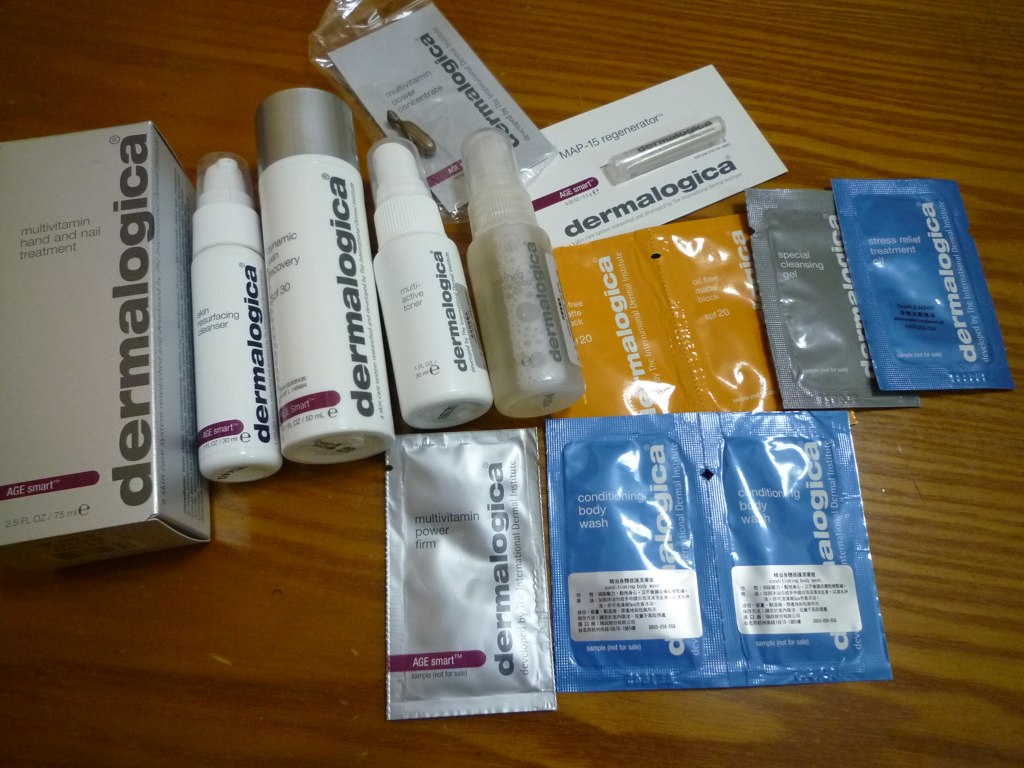In the photograph, an assortment of Dermalogica skincare products are meticulously arranged on a wooden table in an indoor setting. Dominating the left side is a large white box adorned with silver letters spelling "Dermalogica." This box contains a multivitamin hand and nail treatment, with "Age Smart" written in white letters on a purple band near the bottom. Adjacent to the box is a white bottle labeled "Dermalogica Cleanser," also part of the Age Smart collection, featuring a similar purple band.

Next to it is another Age Smart product with a silver cap and a corresponding purple band at the bottom. A smaller spray bottle, branded Dermalogica, sits nearby, followed by a clear bottle containing a transparent liquid, also marked Dermalogica.

The display also includes two yellow pouches, each bearing the Dermalogica logo and indicating a 20 mg content. A silver packet is identified as a special cleansing gel, while a blue pouch labeled "Stress Relief Treatment" showcases "Dermalogica" in white letters against a blue background.

Above these, a small vial noted as a MAP-15 regenerator can be seen. At the bottom of the arrangement, a silver pouch labeled "Multivitamin Power Firm" and two blue packets labeled "Conditioning Body Wash" are present. The latter features a warning label in an unrecognizable language.